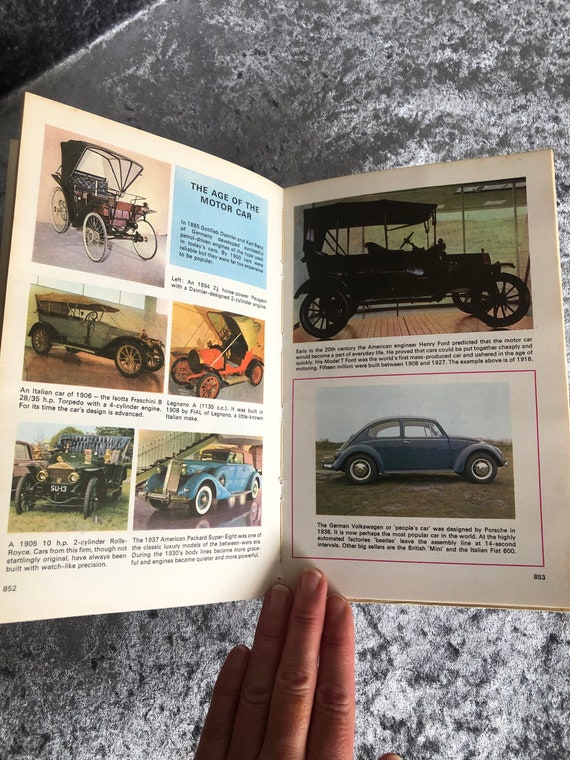In the image, a woman's hand with three visible fingers holds open a small, illustrated booklet against a grayish-white, marbled background, possibly a countertop. The booklet, open to pages 852 and 853, features historical information about motor cars under the title "The Age of the Motor Car,” prominently displayed in a blue box on the left page. The pages exhibit multiple vintage car photos in various colors: blues, blacks, oranges, and greens.

On the left page, there are old car models dating back to the early 20th century (circa 1905 and 1937), and a reference to American engineer Henry Ford. The text includes descriptions such as a meticulous two-cylinder Rolls-Royce, celebrated for its precise craftsmanship. The right page displays more antique cars, including a notable blue Volkswagen Beetle from 1938, often referred to as the "German Volkswagen" or "people's car." Each photograph is accompanied by textual descriptions detailing the make and historical significance of the cars depicted, offering a journey through automotive history.